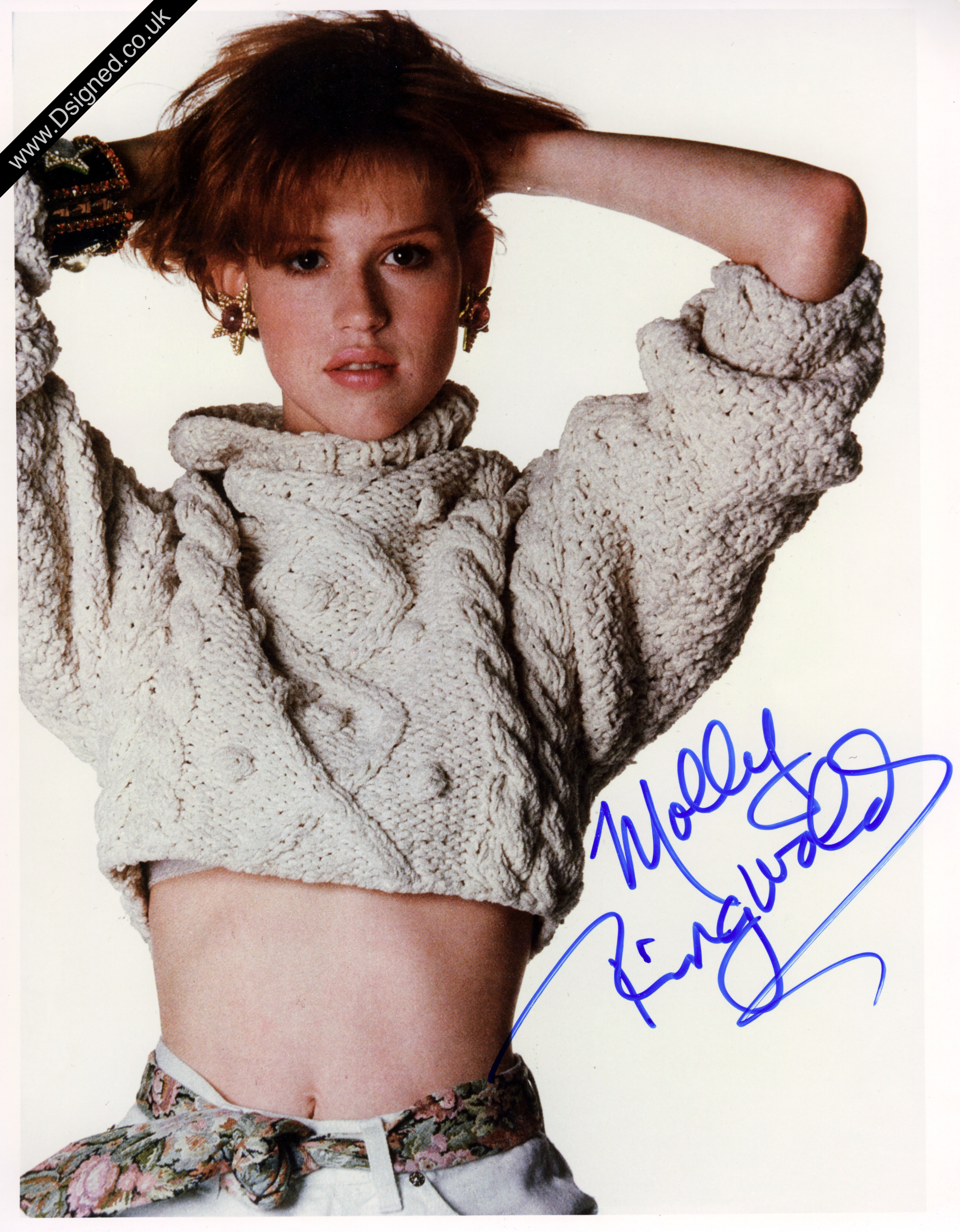This vintage photograph captures actress Molly Ringwald standing against a white background. She is dressed in a high collar, off-white cable-knit sweater that cuts off at the upper belly, revealing her midriff and a glimpse of her white pants. Accentuating her waist is a flowery patterned scarf worn as a belt. Her short, reddish-brown hair is styled in a poofy manner with bangs, and she has her hands positioned behind her head, pushing one sleeve of her thick sweater up over her elbow. Her striking makeup includes lots of eye makeup and peachy lipstick, and she accessorizes with star-shaped earrings. A signature in blue ink, reading "Molly Ringwald," is prominently visible at the bottom right of the image. A black banner with white text "www.design.co.uk" appears diagonally in the upper left corner of the photo.